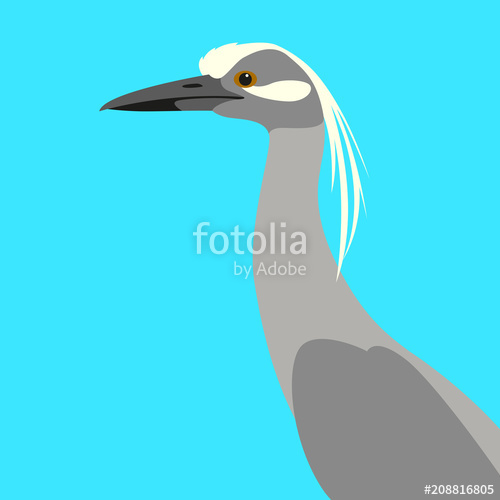This digital, vector-style graphic design features a side profile of a bird on a turquoise background. The bird, bearing a resemblance to a tall, stork-like creature, is predominantly dark and light gray in color, with its head being mainly dark gray and the lower part of the beak in charcoal black transitioning to a lighter gray on top. The beak is notably long, sharp, and pointy. The bird’s eye is black and beady, surrounded by a dark gold and brown ring, punctuated with a white dot in the center. Notably, a flowing white mane, almost mullet-like, extends from the head, drooping down behind the bird and curving around its long neck. The wings are illustrated in dark gray. A watermark in washed-out white text across the center of the image reads "Fotolia by Adobe," accompanied by the small inscription "#208816805" at the bottom right of the bird.